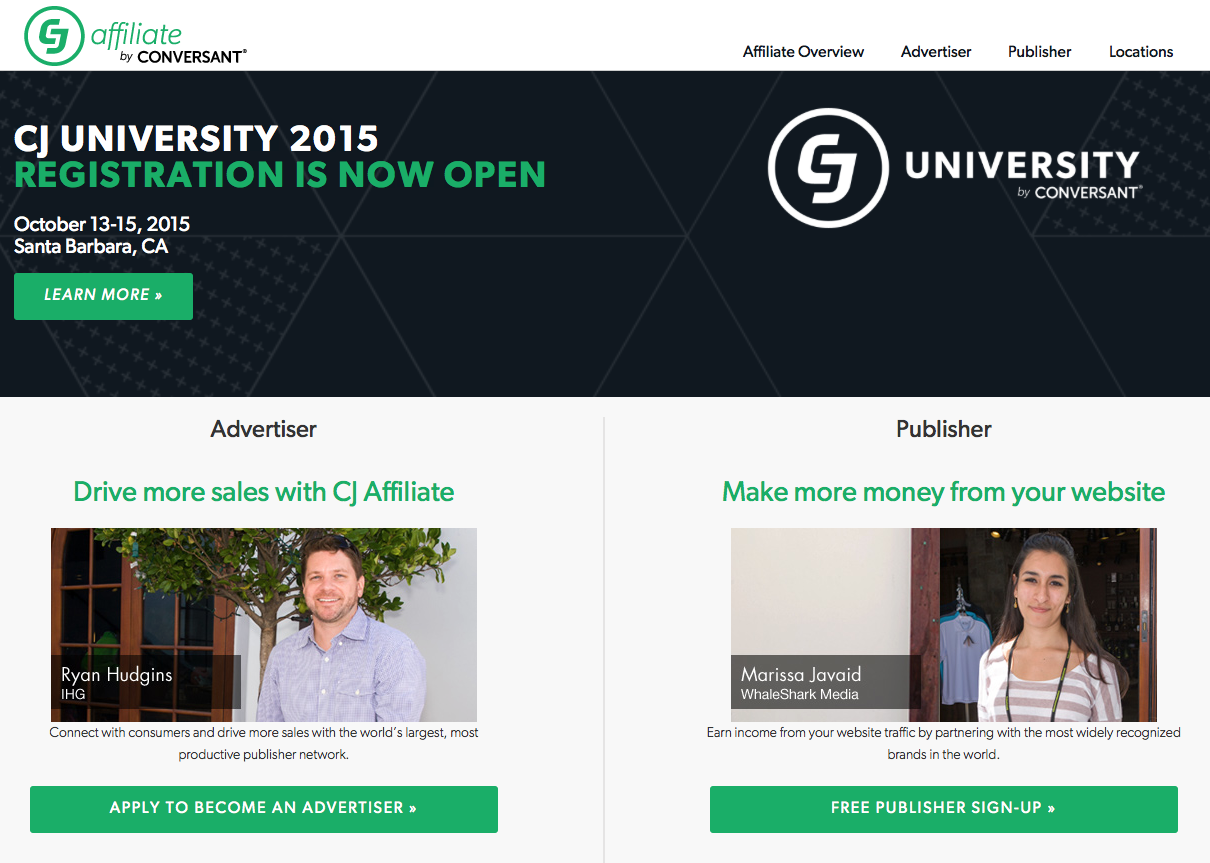**Caption:**

The promotional webpage for CJ University 2015, organized by CJ Affiliate by Conversant, features a detailed layout to attract both advertisers and publishers. At the top, the header displays the "CJ Affiliate by Conversant" logo. A navigation menu on the right includes links such as Affiliate Overview, Advertiser, Publisher, and Locations. The main title, "CJ University 2015," announces that registration is open for the event, scheduled from October 13th to 15th, 2015, in Santa Barbara, California. There's a prominent green button labeled "Learn More."

The Advertiser section encourages businesses to "Drive More Sales with CJ Affiliate" and includes a photograph of Ryan Hudgens from IHG, standing outdoors with a tree and building in the background. The accompanying text highlights the opportunity to connect with consumers through the world's largest, most productive publisher network. A green button invites potential advertisers to "Apply to Become an Advertiser."

The Publisher section urges website owners to "Make More Money from Your Website," featuring an image of Marissa Havig from Whale Shark Media, standing indoors with merchandise in the background. The text emphasizes the potential to earn income by partnering with widely recognized brands. A green button offers a "Free Publisher Signup."

Overall, the webpage is designed to attract advertisers and publishers to join CJ Affiliate and highlights the benefits of the CJ University 2015 event.